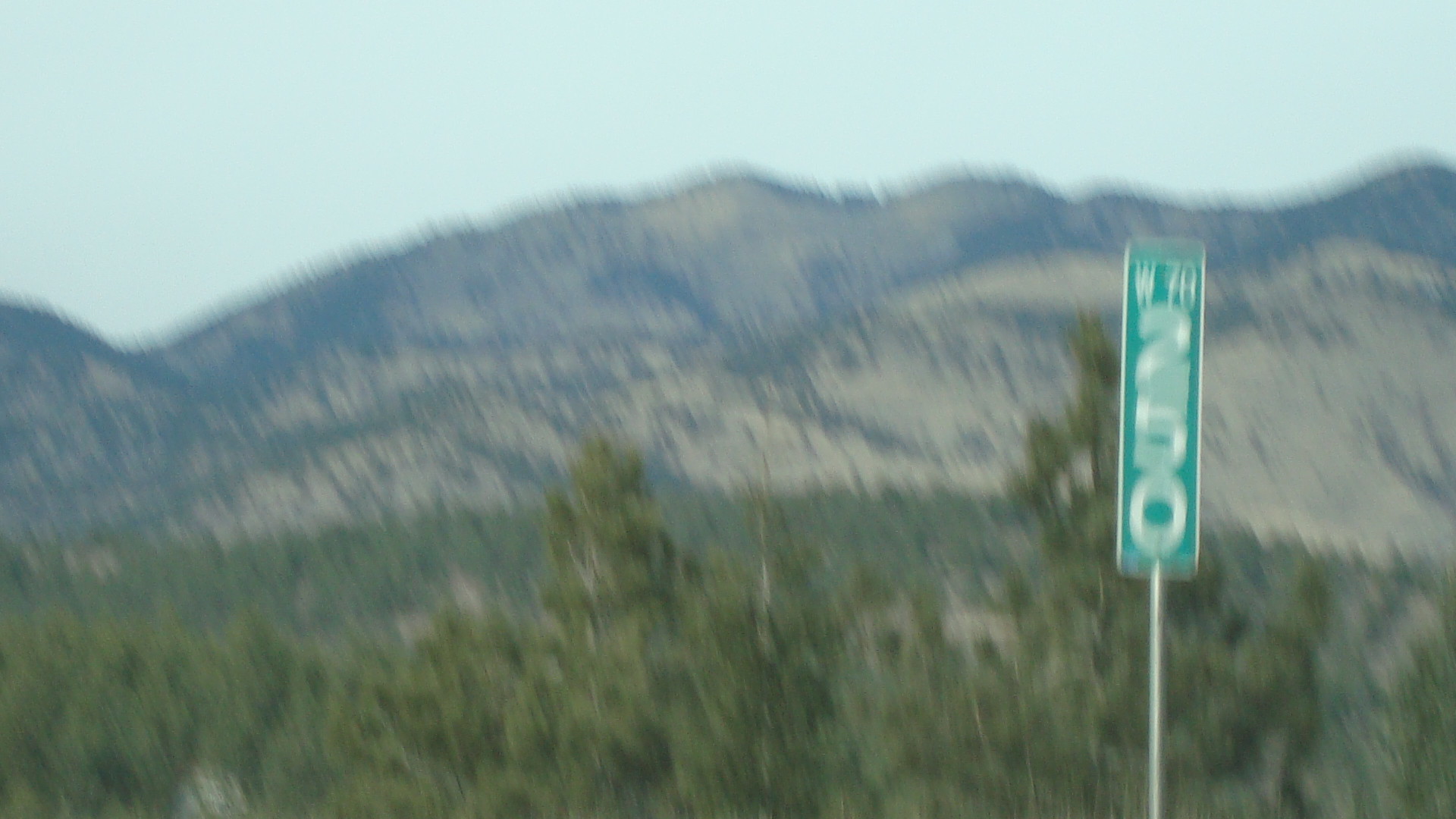This horizontal photograph, although somewhat blurry and likely taken from a moving vehicle, captures a vast daytime landscape with a bright blue sky dotted with minimal white clouds. The background features a range of tall, brown hills speckled with green trees and bushes. Moving towards the foreground, smaller hills similarly adorned with greenery are visible. Dominating the right side of the image is a green highway sign mounted on a slender metal pole. The sign, outlined in white, displays the markings "W70" and "250" in vertically aligned, slightly off-white text.